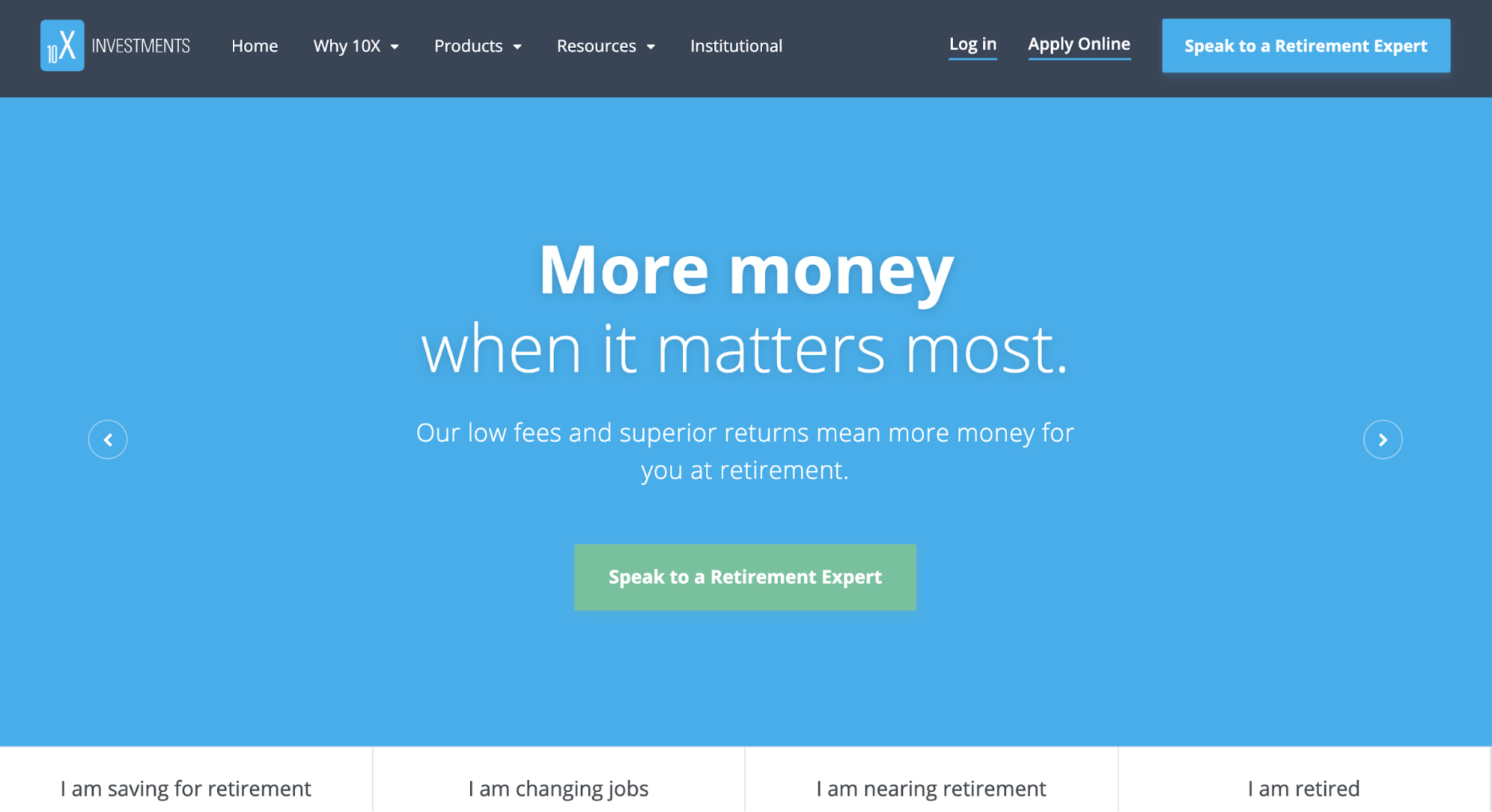This horizontal image appears to be a screenshot of a website's interface, likely accessible via smart devices or computers. The website features a dark gray to black navigation bar at the top. On the left side of this bar, there is a small blue icon with "X" and "10" inside it, labeled "Investments" in white text. Other navigation options include Home, Y, 10X, Products, Resources, and Institutional, listed in a row.

Towards the right end of the bar, there are links to log in, apply online, and a blue button labeled "Speak to a Retirement Expert" in white text. Below the navigation bar, a large blue banner prominently displays the slogan "More Money" in bold white text, followed by "When it Matters Most" in regular white text, and "Our Low Fees and Superior Returns Mean More Money for You at Retirement" in a slightly smaller font.

On either side of this banner, there are arrows for navigating through content. Beneath the main headline, a green button with white text invites users to "Speak to a Retirement Expert." At the bottom of the page, a series of clickable options in black text are presented: "I am Saving for Retirement," "I am Changing Jobs," "I am Nearing Retirement," and "I am Retired."